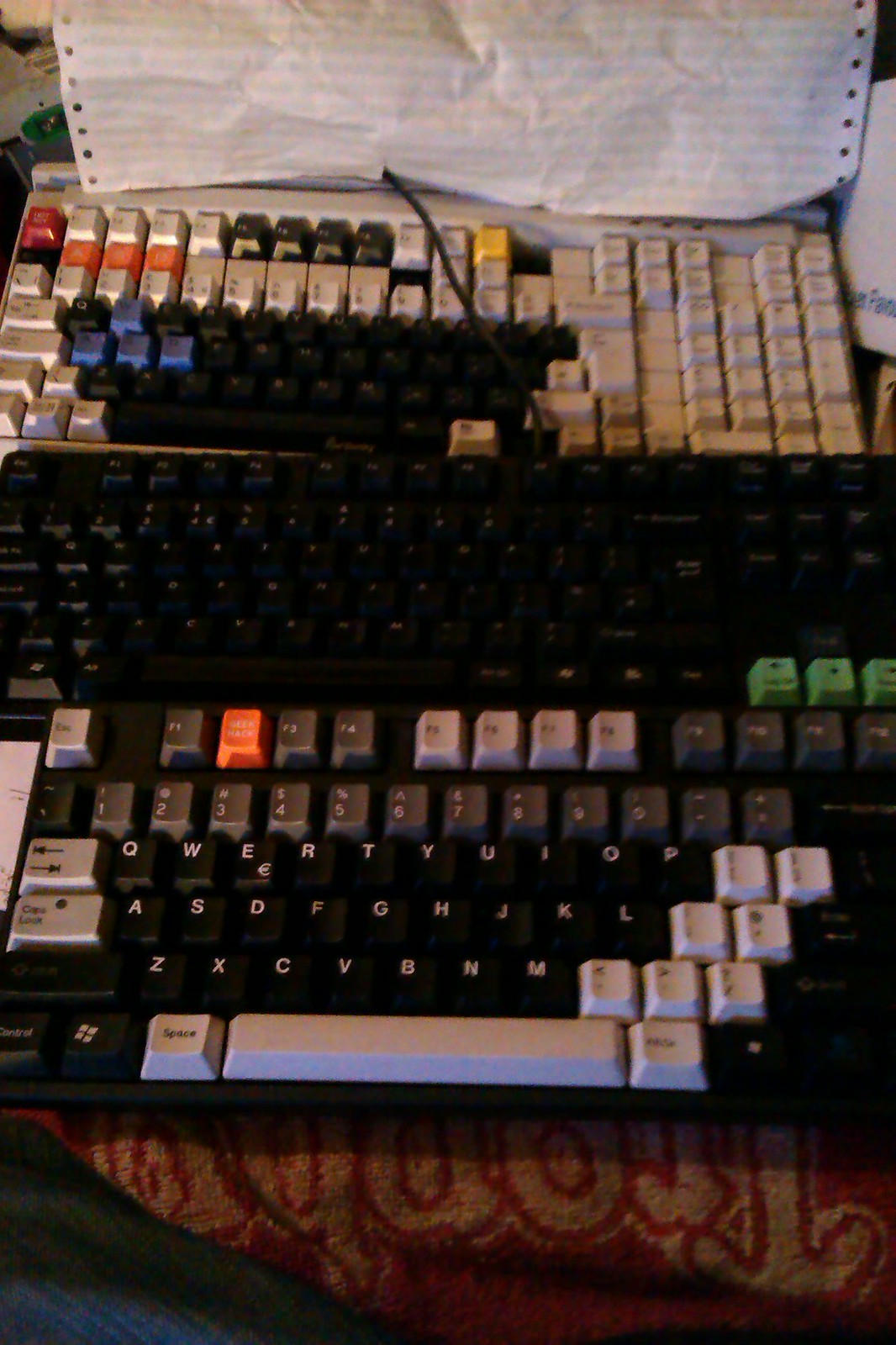The image showcases three custom-made, non-standard keyboards arranged from top to bottom in a low-quality photo. The bottom keyboard is predominantly black with distinctive white keys, including the space bar and symbols for greater than, less than, and brackets. The top row numbers are dark gray, and there's a striking orange F2 key alongside a gray-white ESC key. The middle keyboard is fully black, with the only color variation being three green arrow keys. The top keyboard, in contrast, is mostly an off-white ivory color, featuring black letter keys, a black space bar, red ESC, and a mix of blue, yellow, and orange keys dispersed throughout, including blue WASD keys. A wrinkled piece of paper, resembling fax paper with stripes and holes, partially intrudes into the frame. All three keyboards rest on a surface covered with a dark red and beige material, adding to the eclectic and somewhat cluttered backdrop.